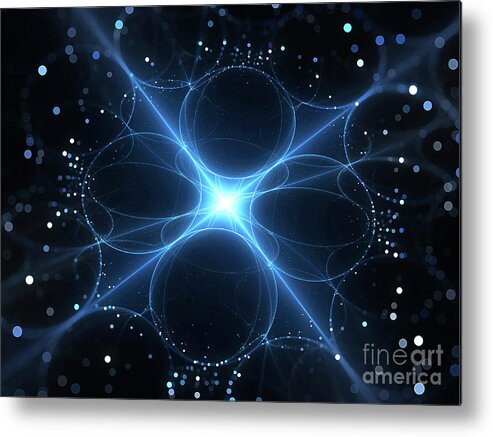This meticulously created digital art piece, which could be CGI, features a central bright white light surrounded by a subtle gradient of light blues. Emerging from this nucleus are piercing light rays that emanate in multiple directions: up-right, down-right, up-left, and down-left, forming an X pattern. The image is set against a black background, which enhances the starkness of these beams. Encasing the central light are four distinct circles positioned to the left, right, above, and below, each with varying intensities and designs of black. The top and bottom circles have denser black centers, while those on the sides have elongated oval black shapes. These circles are connected by a diamond-shaped array that fractures the radiance outward.

The entire composition is bordered by a multitude of tiny white and light blue dots scattered across the four triangular sections created by the light beams, resembling stars or dew drops catching sunlight. Notably, more of these concentrated dots appear in the middle left, middle right, and bottom center sections. Adding depth, a shadow effect is visible along the right and bottom edges, giving a slightly 3D feel to the rectangular image, which measures approximately 3 inches by 3.5 inches. The bottom right-hand corner discreetly features the text "Fine Art America" in gray, with "art" and "America" in slightly bolder print.